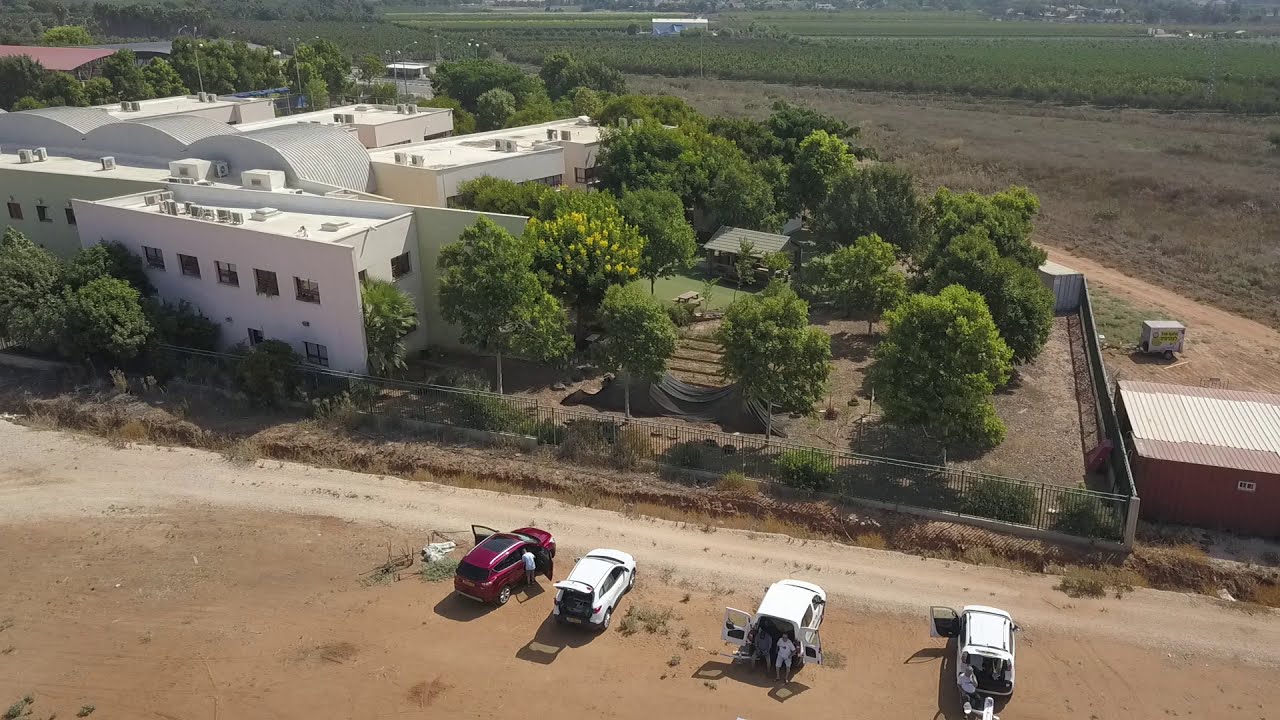This aerial color photograph, captured in landscape orientation, showcases a picturesque, lush green field intersected by a distinctive brown dirt road. In the foreground, a sandy patch hosts four parked vehicles—three white and one red—with their trunks open, with a few people lounging around. To the left of this sandy area lies a fenced-off section containing several green trees and a verdant lawn, flanked by a cluster of white, two-story buildings which resemble research facilities or laboratories. Adjacent to the buildings, there's a group of white circular structures, akin to greenhouses, surrounded by additional green pastures. Beyond the foreground, the landscape stretches into farmlands with smaller buildings dotted in the distance.